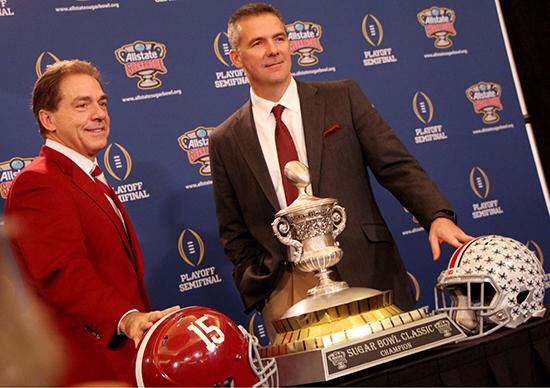The image depicts two distinguished gentlemen standing together at a football-related event, likely within the context of a public ceremony or celebration. They are dressed in formal attire: the man on the left wears a striking red suit and white tie, while the man on the right sports a brown suit, red tie, red handkerchief, and light brown pants. Both men have their hands on football helmets placed before them. The man in the red suit rests his hand on a red helmet adorned with the number 15 and a white stripe, while the man in the brown suit touches a white helmet decorated with black stars and red and blue stripes. Positioned between them is a trophy with "Sugar Bowl Classic Champion" engraved on its base. The backdrop of the scene is a deep blue banner featuring various insignias, including miniature trophies and footballs, with the words "playoff semi-final" displayed prominently. Both gentlemen are smiling subtly and looking slightly away from the camera.